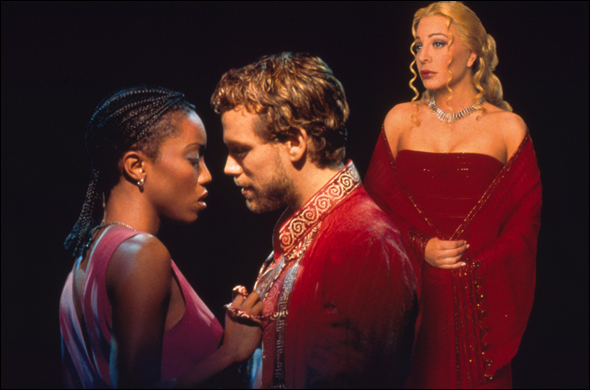In the striking photograph, three individuals stand against an all-encompassing black background, giving the appearance that they are floating in a void. On the far left is a woman in a sleeveless purple dress. Her shoulder-length black hair is styled in braids, and she accessorizes with silver hoop earrings and what might be a bracelet on her wrist. Her right hand rests on the chest of the man standing in the center, slightly pulling at the fabric of his elaborately designed red coat, which features a tall collar adorned with intricate gold embellishments. This man, who is facing her, has a blonde beard and medium-length curly hair.

To the right of the man and positioned slightly to the back, another woman stands. She is dressed in an elegant, strapless red dress accompanied by a matching red shawl. Her long blonde hair cascades down, and a silver necklace graces her neck. Her posture is composed, with her hand resting in front of her, and she gazes forward, adding a contemplative air to the scene. The intricate details of their attire and the dynamic positioning of their bodies against the stark, black void create an evocative and compelling image.